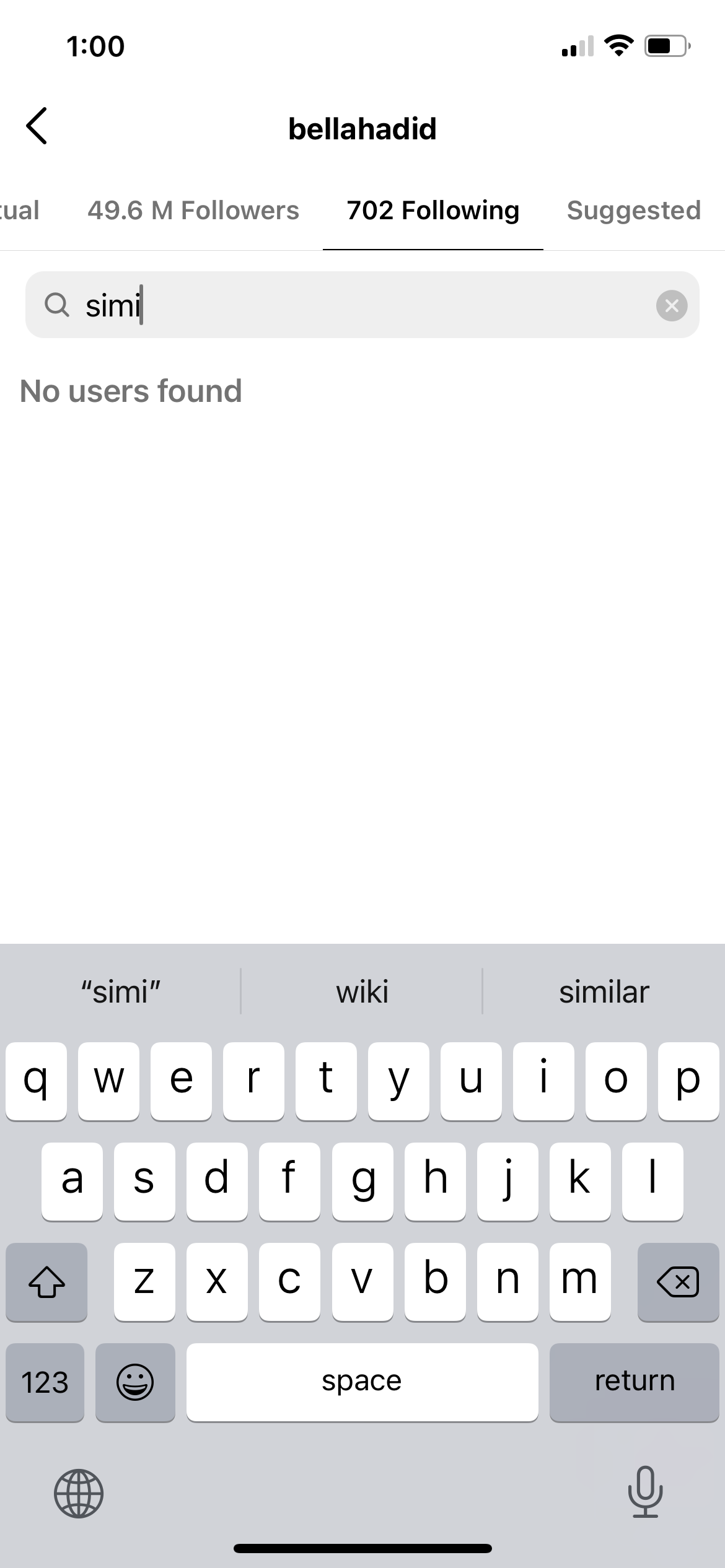The image displays a mobile phone screen, specifically an iPhone, with prominent details indicating various on-screen elements and activities. At the top of the screen, the time is noted as 1:00 PM, with the status bar showing two bars of internet signal, full Wi-Fi connectivity, and approximately two-thirds battery life remaining. There's also a back arrow icon for navigation.

Dominating the center of the screen is a social media profile under the username "Bella Hadid," evident from the profile information displayed. The account boasts an impressive following of 49 million followers, alongside a count of 702 accounts that Bella Hadid is following. The user appears to be actively engaging with this profile, observed from the text entry in a search box where they have typed "S-I-M-I." This input suggests the user is searching for a follower or a friend within Bella Hadid’s following list. However, no results appear to match the search query, indicating that Bella Hadid is not following anyone with a username starting with "S-I-M-I."

At the bottom of the screen, the familiar iPhone interface is visible, including typical icons and functionalities, underscoring a standard user experience.